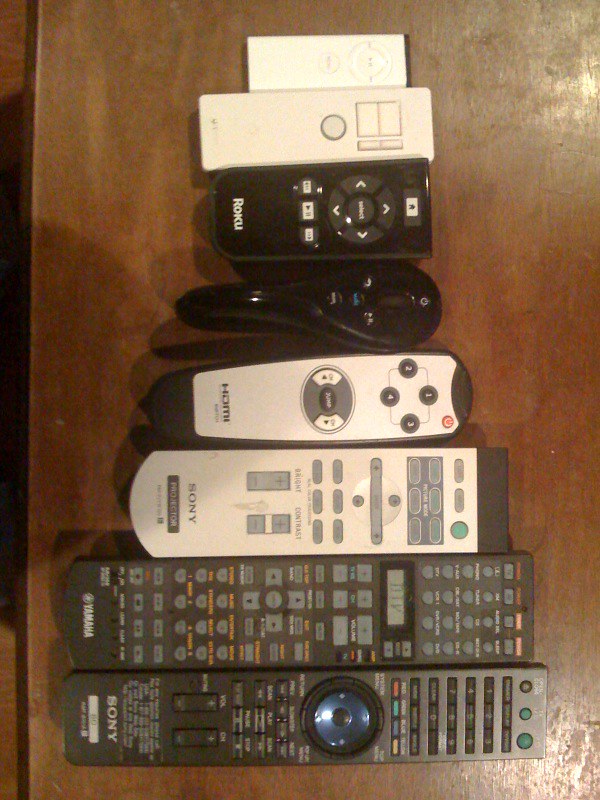This photograph captures eight remote controls meticulously arranged on a dark brown wooden table. The remotes are aligned from largest to smallest, with the largest at the bottom and the smallest at the top. Each remote is positioned with its infrared sensor facing to the right.

The largest remote, at the bottom, is a classic Sony TV remote, recognizable by its central navigation panel and copious buttons. Above it is a Yamaha TV remote, also large and filled with numerous buttons. Next up is another Sony remote, this one off-white with gray buttons, likely for controlling a projector given the "bright contrast" label.

The following remote is white with "HDMI" text on it, suggesting its use for an audio-visual device. Above it is a uniquely shaped black remote resembling a tennis racket, featuring a handle and a few unmarked buttons.

The subsequent device is a black Roku remote, marked clearly in white letters. Following that is a small white remote with minimal buttons, likely for basic functions. At the very top lies the smallest of the lot, another simple white remote with just a power and play button.

All these remote controls vary significantly in design, purpose, and age, providing a fascinating glimpse into the evolution and diversity of remote control technologies.